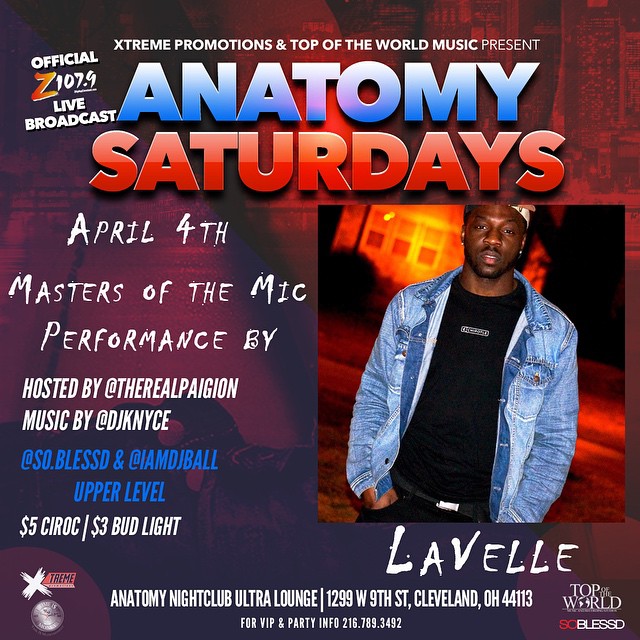The image is a digital advertisement for a music performance at Anatomy Nightclub Ultra Lounge, located at 1299 West 9th Street, Cleveland, Ohio 44113. The poster, featuring a purple to red gradient background, prominently highlights "Anatomy Saturdays" with "Anatomy" in blue and "Saturdays" in red. Presented by Extreme Promotions and Top of the World Music, it announces an official Z107.9 live broadcast on April 4th, with a "Masters of the Mic" performance by Lavelle, depicted as a black man in a red or blue jacket, black t-shirt, and black pants. The event is hosted by The Real Pagean, with music by DJ KNYCE, So Blessed, and I Am DJ Ball. The upper level offers $5 Ciroc and $3 Bud Light. For VIP and party information, contact 216-789-3492.